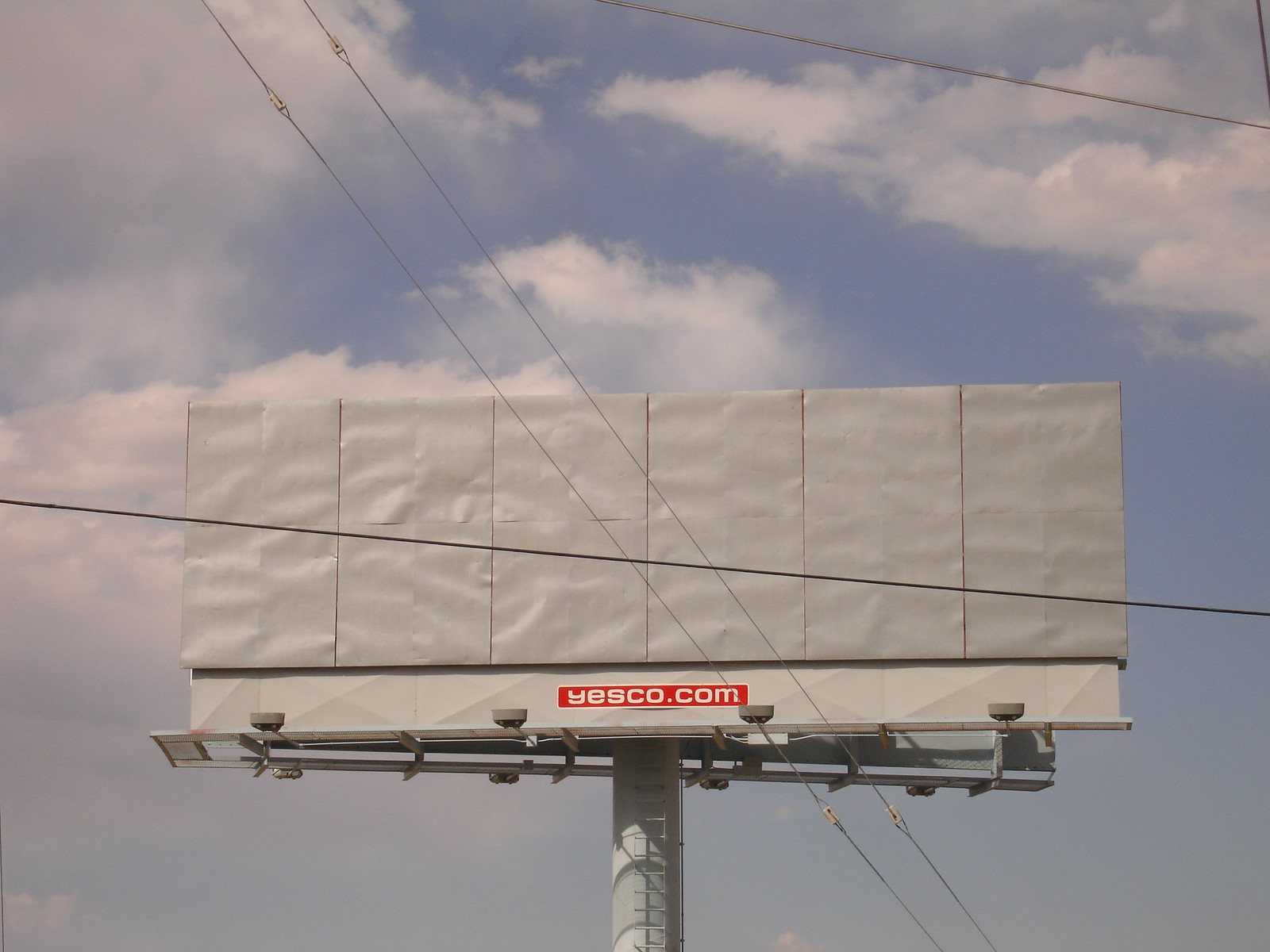The image is a horizontally-oriented color photograph, capturing a large billboard against a soft, cloudy blue sky. The post holding up the billboard is cut off at the bottom center of the image, and its light gray structure features a set of ladders or stairs ascending towards the sign. The billboard itself bears the text "yesgo.com" on a small red strip positioned at the bottom. The main face of the billboard is covered with six vertical strips of paper, creating an obscured effect. 

Crisscrossing the billboard are several wires: one horizontal wire tilts downward through the center of the image, while two other wires stretch diagonally from the top left corner towards the bottom right corner. A final wire runs from the top center to the top right of the billboard. The background features a tranquil, partly cloudy sky with fluffy clouds, providing a serene backdrop to the industrial structure. The overall color scheme of the billboard and its coverings is a muted grayish-beige.